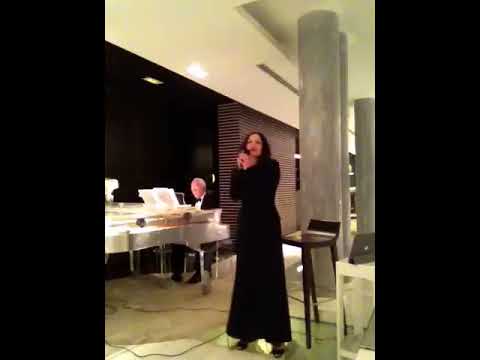In this photo, a young woman in a long black formal dress is center stage, holding a microphone close to her mouth as she sings to an unseen audience. Her cupped hands before her face emphasize her vocal performance. In the background to her left, an older man with gray hair, dressed in a tuxedo, is playing a white piano. The setting appears to be a formal venue, possibly a hotel lobby, characterized by pillars extending into the background. Behind the woman, there is a high bench that appears to be holding something, possibly a computer. Additionally, there’s a chair visible and a plaque on a nearby table, adding to the formal and elegant atmosphere of the scene.